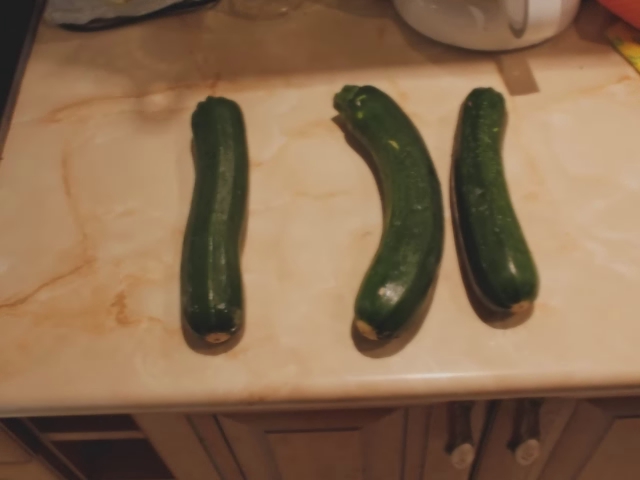This image captures a kitchen scene with a dimly lit ambiance imparting a yellow hue. At the focal point, three green cucumbers of varying sizes and shapes lie side by side on an off-white granite countertop with tan veining. The cucumbers have visible marks and dents, and their shapes vary: the middle cucumber curves like a banana, while the ones on either side are straighter but still display gentle bends. Below the countertop, a brown wooden cabinet is partially visible, adding a rustic element to the scene. In the background, a white pot sits on the countertop, and faint shadows play across the surface due to the soft, diffused lighting. The overall impression is that of a casual, candid photograph, likely taken to highlight a fresh purchase from a market.